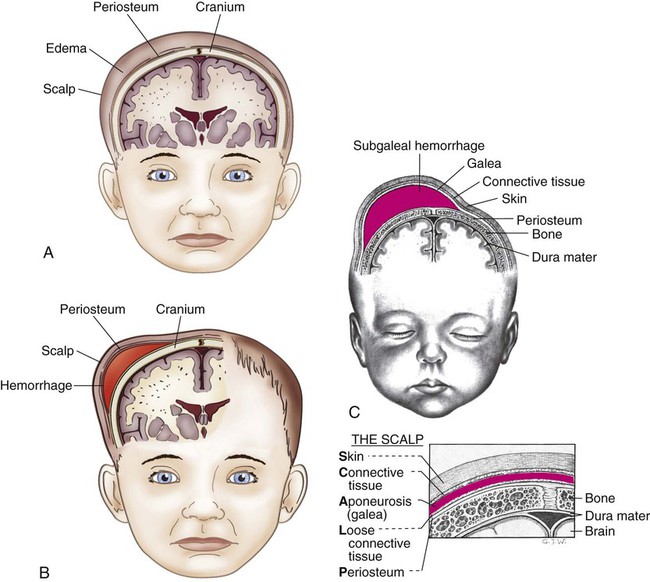The image consists of three detailed anatomical illustrations labeled A, B, and C, showcasing the cross-section of a child's head. These illustrations are meticulously labeled for educational purposes, likely aimed at medical students. The diagrams highlight various layers and structures, including the scalp, skin, connective tissue, periosteum, cranium, edema, dura mater, and the brain. Figure A features a colorful depiction of a child's head, revealing the scalp and underlying layers such as the connective tissue and dural areas, emphasizing how these parts interact. Figure B delves deeper into the anatomy, with a further sectioned view exposing more detailed layers and potential areas of hemorrhage. Figure C transitions into a black-and-white illustration, presenting the child with closed eyes and mouth, while further annotating specific regions including the galea aponeurotica, loose connective tissue, and more magnified sections to provide an enhanced view of critical structures. The child's head illustrations also depict brown hair, blue eyes, and Caucasian skin, encompassing varied perspectives to facilitate comprehensive anatomical understanding.